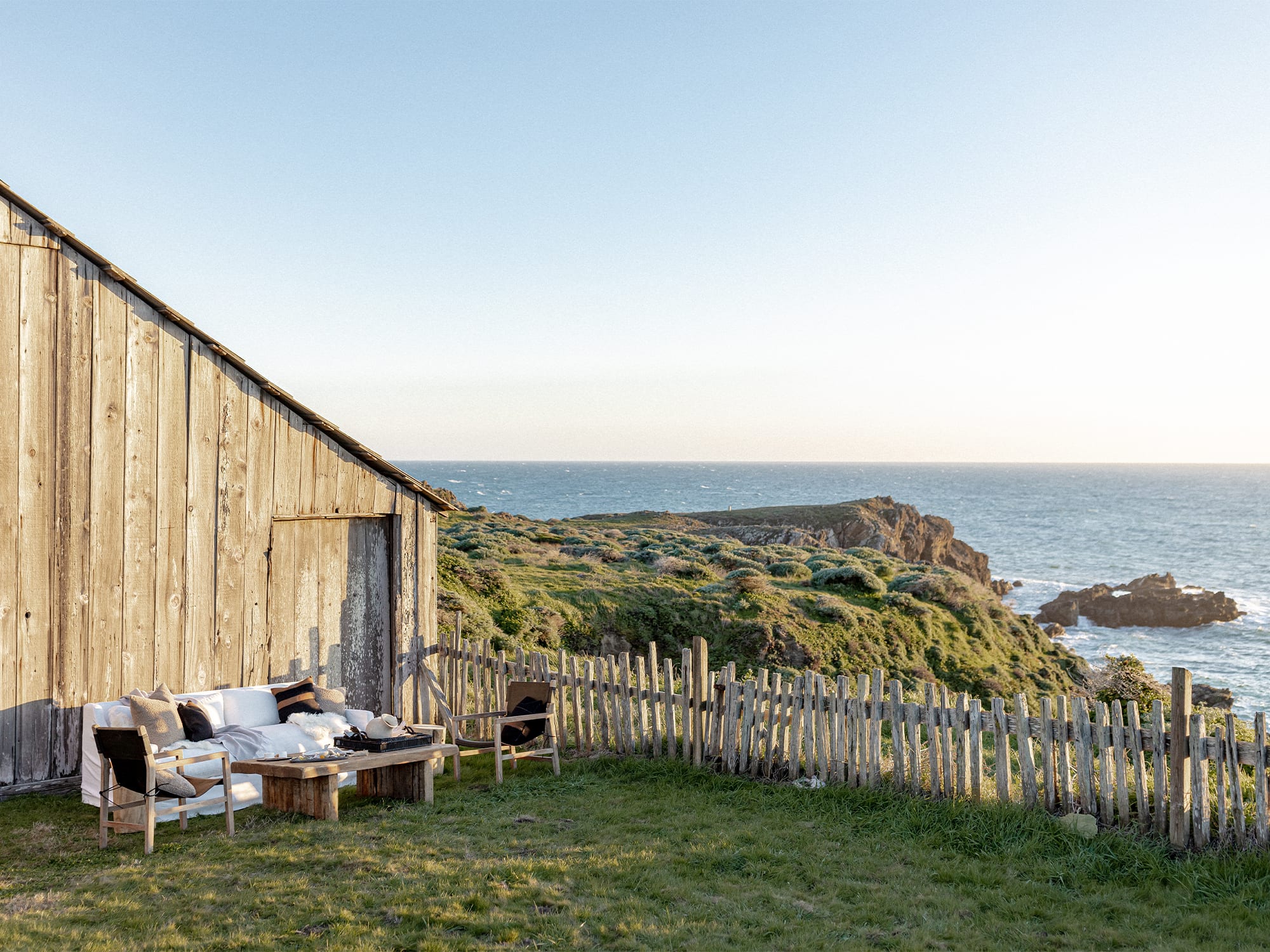Set against a serene coastal backdrop, the image showcases a wooden hut on the left side of a grassy hill, extending downward from left to right. The hut, made from light, weathered wood, features a door on the right and a small outdoor seating area in front. The seating area includes a white couch with brown pillows, a small brown table, and two brown wooden chairs on either side of the table. A wooden fence with small vertical slats extends to the right of the door, blending seamlessly with the natural surroundings. The hill, covered in short green grass, becomes increasingly rocky and jagged as it stretches toward the sea, visible in the background. The calm sea has gentle waves and scattered rocks, with a sky that transitions from a serene blue at the top to a mix of lighter hues and a soft orange near the horizon, suggesting either an early morning or evening setting. This idyllic scene evokes a peaceful, picturesque coastal landscape, reminiscent of Ireland’s scenic coastline.